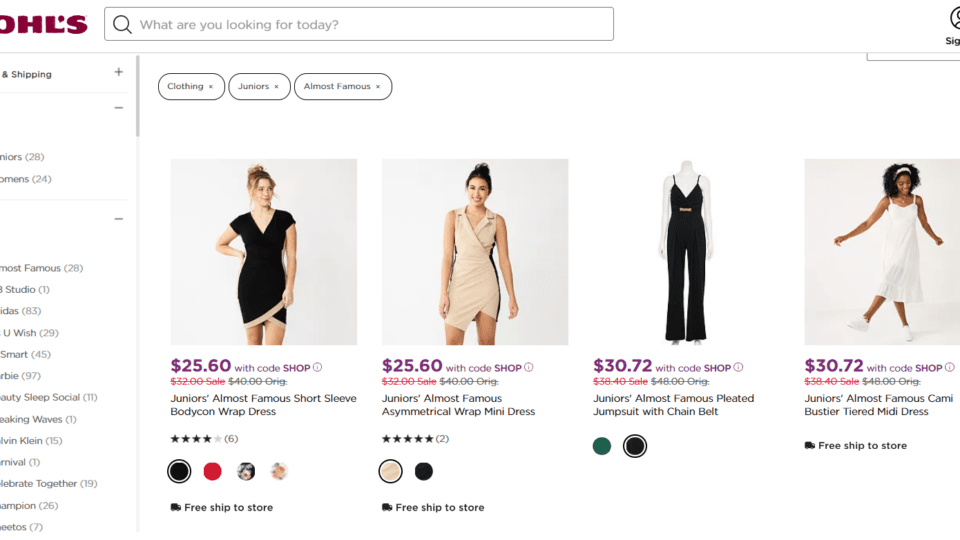On a popular shopping website, likely Kohl's, the top banner displays a partially visible maroon logo reading "OHL,S," along with a search bar prompting, "What are you looking for today?" in grey. To the far right, there's an option to sign in.

The search results for "clothing juniors almost famous" showcase four different pieces of clothing:

1. **First Item**: A Caucasian woman with blond hair styled in a bun is modeling a black V-neck dress that falls above her knees. The dress features a sandy-colored stripe around the hem and has short sleeves. Priced at $25.60 during a sale, this Junior's "Almost Famous" short sleeve bodycon wrap dress is available in multiple colors. The item also offers free shipping to the store.

2. **Second Item**: A woman with tanned skin and dark hair in a bun is wearing a sleeveless sandy-colored wrap dress with black stripes running down each side of the body. This dress, priced similarly at $25.60, includes a collar and also comes in a black and sandy color combination. It has received a five-star rating.

3. **Third Item**: Displayed on a mannequin, this item is a V-neck spaghetti strap jumpsuit with long legs, available in black. This piece is priced at $30.72 and comes in a green variant as well.

4. **Fourth Item**: A Black woman with shoulder-length hair and a cheerful smile is shown kicking one leg in the air while wearing white sneakers and a long, white, mid-calf dress with strappy straps. This dress is priced at $30.72. 

These detailed descriptions highlight the variety and style of clothing available in the searched category.